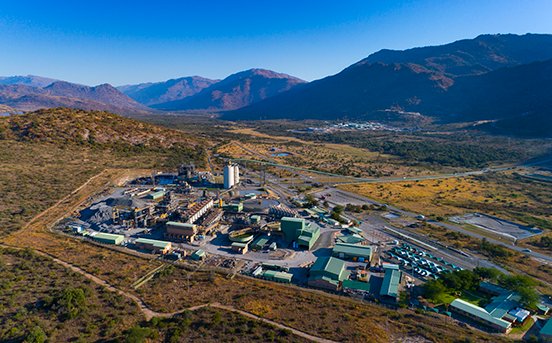This aerial photograph, possibly taken by a drone or helicopter, captures a detailed view of an expansive facility nestled within a large valley that slopes into a mountainside to the right. Dominating the image are the facility's rooftops, with some displaying a distinct green hue. It's evident that the facility is a hub of activity, as the parking lot contains several cars. Surrounding the facility, the untouched shrubbery and natural landscape contrast with the built environment.

Beyond the facility, sprawling green grasslands extend toward the horizon. The image reveals well-defined roads encircling the area, suggesting accessibility and connectivity. In the distance, the silhouette of a larger city emerges, its buildings faintly visible against the backdrop of picturesque, cloudless blue skies and majestic mountain ranges. Notable are several white cylindrical buildings that stand out within the facility, hinting at an industrial or work site, adding to the complexity and utility of the scene.